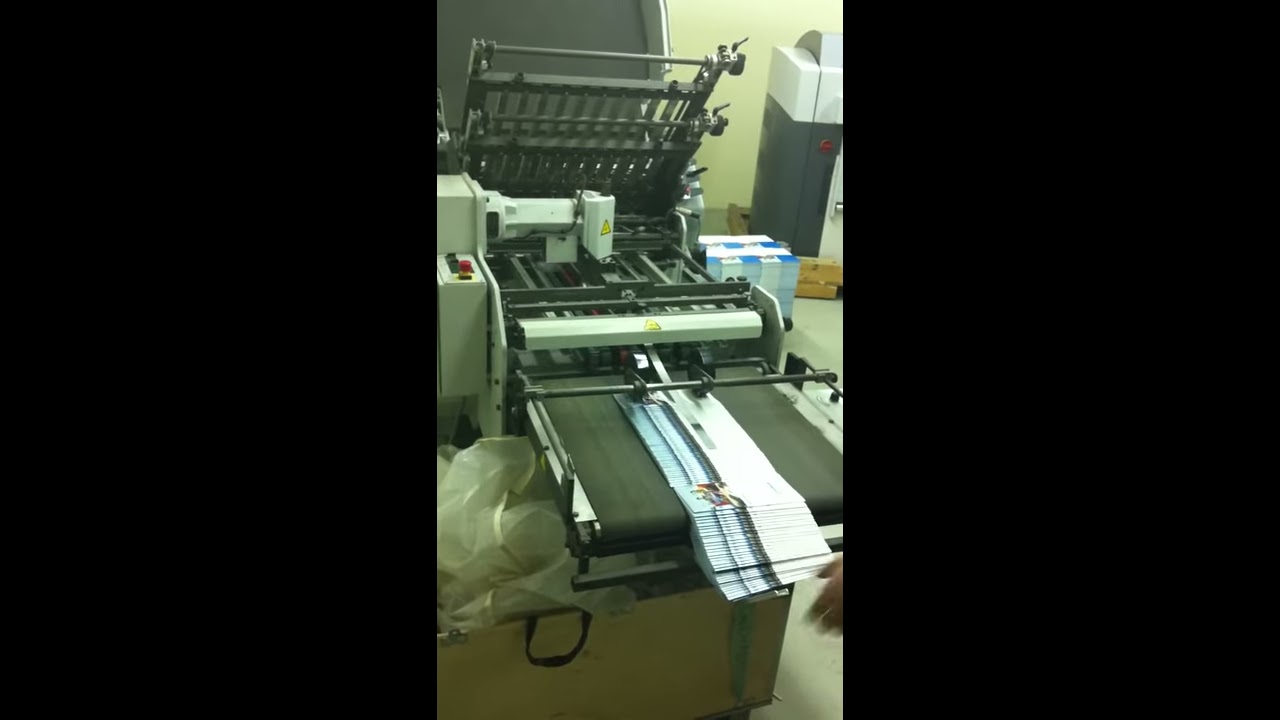This detailed photograph showcases a metallic printing machine in an indoor setting, captured in portrait orientation. The machine, largely gray and silver with a few elements in cream, is equipped with various parts, including a small black conveyor belt at the end. Emerging from the conveyor belt are paper posters or booklets, indicating the machine’s function as a printing press, likely for small-scale newsletters or brochures. A caution sticker, a yellow triangle with a black border, is visible on the machine, highlighting potential operational dangers. A red switch and operational buttons are also noticeable on the left side of the machine. The image partially shows a human hand near the conveyor belt, hinting at manual intervention but the rest of the person remains out of the frame. Surrounding the machine, the floor is cluttered with stacks of paper, cardboard boxes, and other items, adding to the industrial ambiance. The photograph features vertical black strips on either side of the frame, and despite the detailed machinery in the center, about two-thirds of the image fades into blackness, creating a stark contrast with the illuminated equipment.